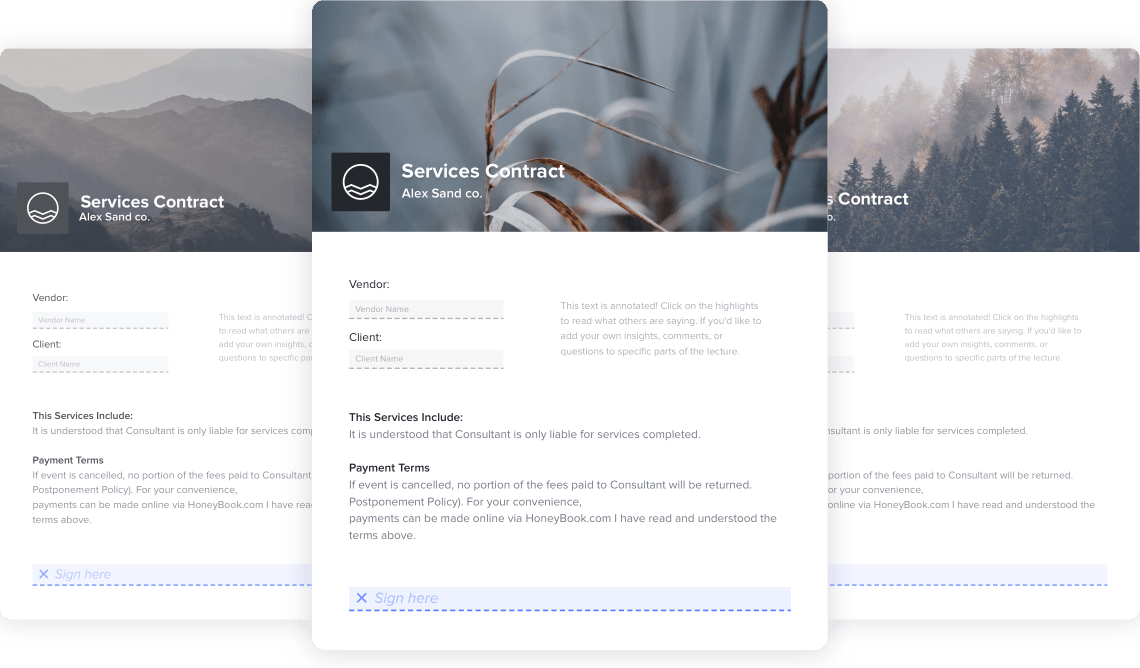This composite image comprises three distinct nature scenes arranged artistically, with two images in the background and a third image overlaid in the center. Each image captures different elements of nature, presented in a calming brown and gray color palette.

The first image, positioned in the background, features softly muted hills that are slightly grayed out, creating a tranquil ambiance. Superimposed text on this image reads "Services Contract Alex Sandco" in white font, accompanied by a gray square containing a white circle. Below, there are labeled boxes for "Vendor" and "Client," currently blank. The image also includes multiple lines of gray text in black font, addressing various terms of the service contract:
- "The service includes it is understood that consultant is only available for services."
- "Payment terms: If the event is canceled, no portion of the fees paid will be returned."
- A box for signatures to affirm understanding of the terms.

The second image, placed partially behind but more to the foreground of the first, highlights a close-up shot of a brown plant set against a similarly grayish background. This section also displays text confirming the "Services Contract for Alex Sandco," reiterating the vendor and client boxes, and providing a detailed paragraph allowing for comments and insights:
- "This text allows you to read what others are saying. It's a place to add your own insights or comments."
- "The service includes if understood this consultant is only viable for services completed."
- "Payment terms: If the event is canceled, no portion of the fees paid will be returned."
- "Postponement policy: For your convenience, payments can be made online via honeybook.com."
- An affirmation section "I have read and understood the terms above," followed by a signature box.

The third and final image, centrally overlaid, showcases a serene forest scene viewed through a brown and gray lens. It mirrors the previous textual content:
- Confirmation of the service contract.
- Labeled boxes for "Vendor" and "Client."
- A comprehensive explanation of the service terms, postponement policy, and online payment instructions.

Overall, this composite image not only illustrates the beauty of nature but also serves as a structured and detailed depiction of a contract for services offered by Alex Sandco, complete with areas for comments, signatures, and terms understanding.